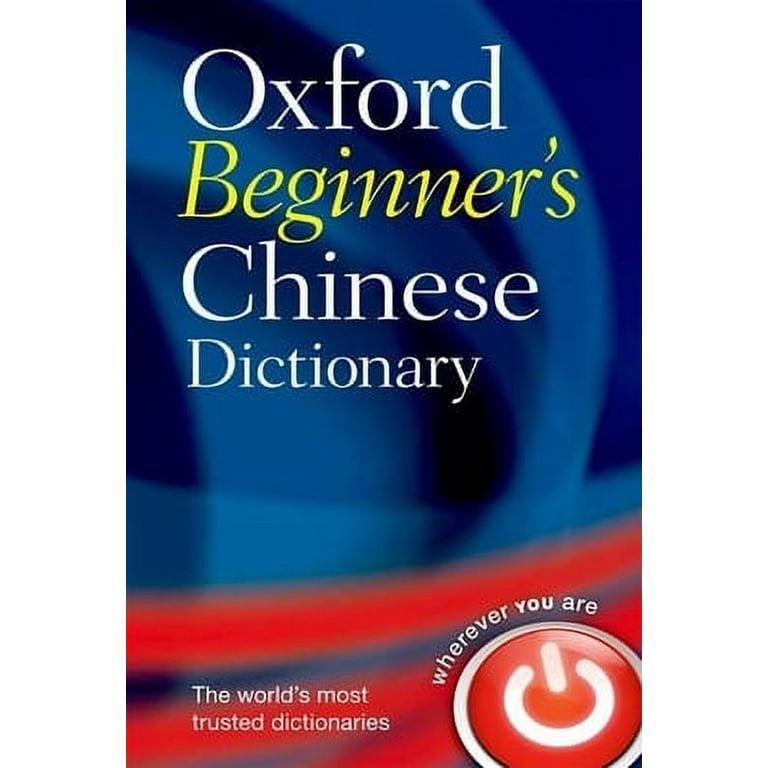The image displays the cover of a book titled *Oxford Beginner's Chinese Dictionary*. The background is primarily blue with dynamic, lighter blue swashes that add a sense of movement to the cover. The title elements "Oxford" and "Chinese Dictionary" are written in white, with "Beginner's" emphasized in yellow italics. Below the blue background, the lower portion of the cover transitions into red tones with sweeping swishes from left to right, creating a vibrant contrast with the upper blue section. On the left side of this red lower section, white text reads "The World's Most Trusted Dictionaries," while on the right, next to a shiny red power button symbolizing the word "ON," is the phrase "wherever you are," with the "U" in bold to add emphasis. This cover, which appears to be a digital rendering much like the first page of a PDF copy, gives a comprehensive and visually engaging introduction to the Oxford Beginner's Chinese Dictionary.